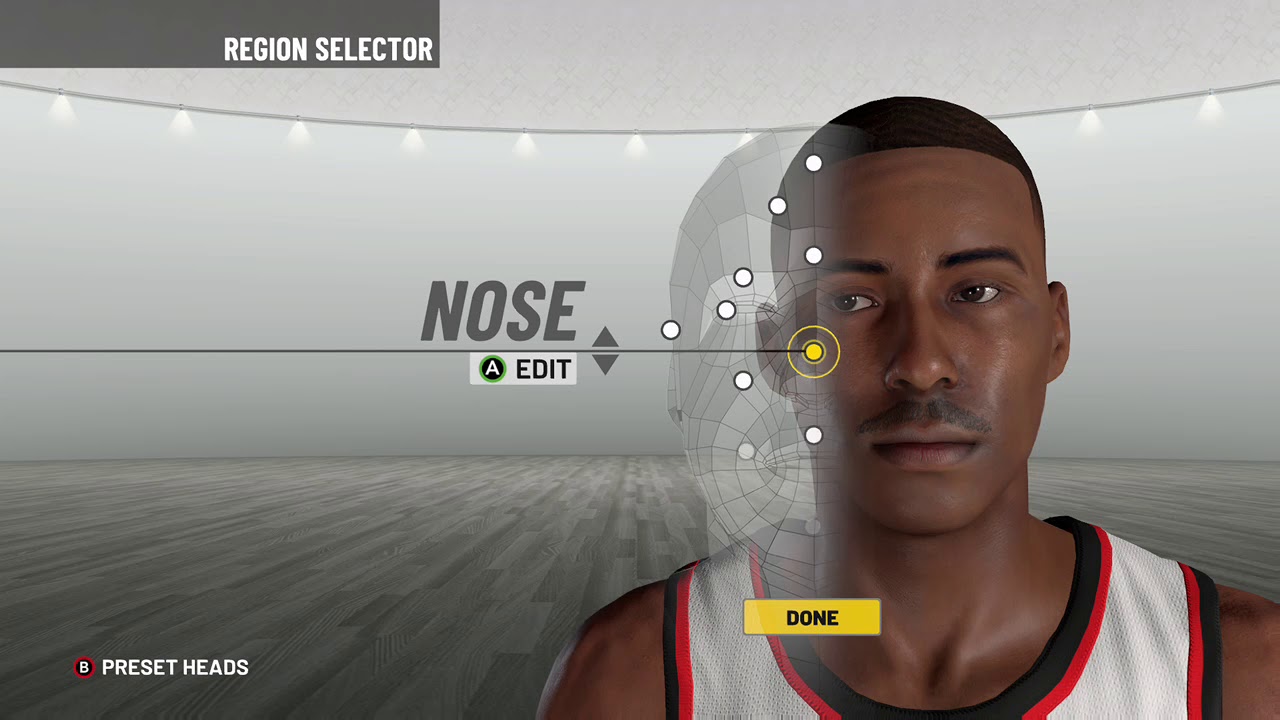The image depicts an African-American man with very short, almost shaved black hair, accompanied by dark black eyebrows, dark brown eyes, and a faint mustache. He is wearing a sleeveless basketball tank top, trimmed in black around the collar and orange around the upper sleeves and neckline. 

The background is a light gray, with a dark gray banner on the left side that reads "Region Selector" in white text. There is also a string of lights or similar detail running across the top of the image, though its purpose is unclear. 

In the middle of the image, a fine gray line extends from the left to the man's right cheek, where it connects to a yellow circle surrounded by small white dots. This line is labeled "Nose" in dark gray text, suggesting that this is an area that can be edited. Directly below this, a banner with "Edit" in dark gray text appears, accompanied by a black circle with a white "A" inside it. 

At the bottom of the image, a yellow banner with "Done" written in dark brown text indicates the option to finalize the edits. Additionally, a red circle on the far left containing a white "B" accompanies the text "Preset Heads" in white, potentially offering pre-set facial features or shapes.